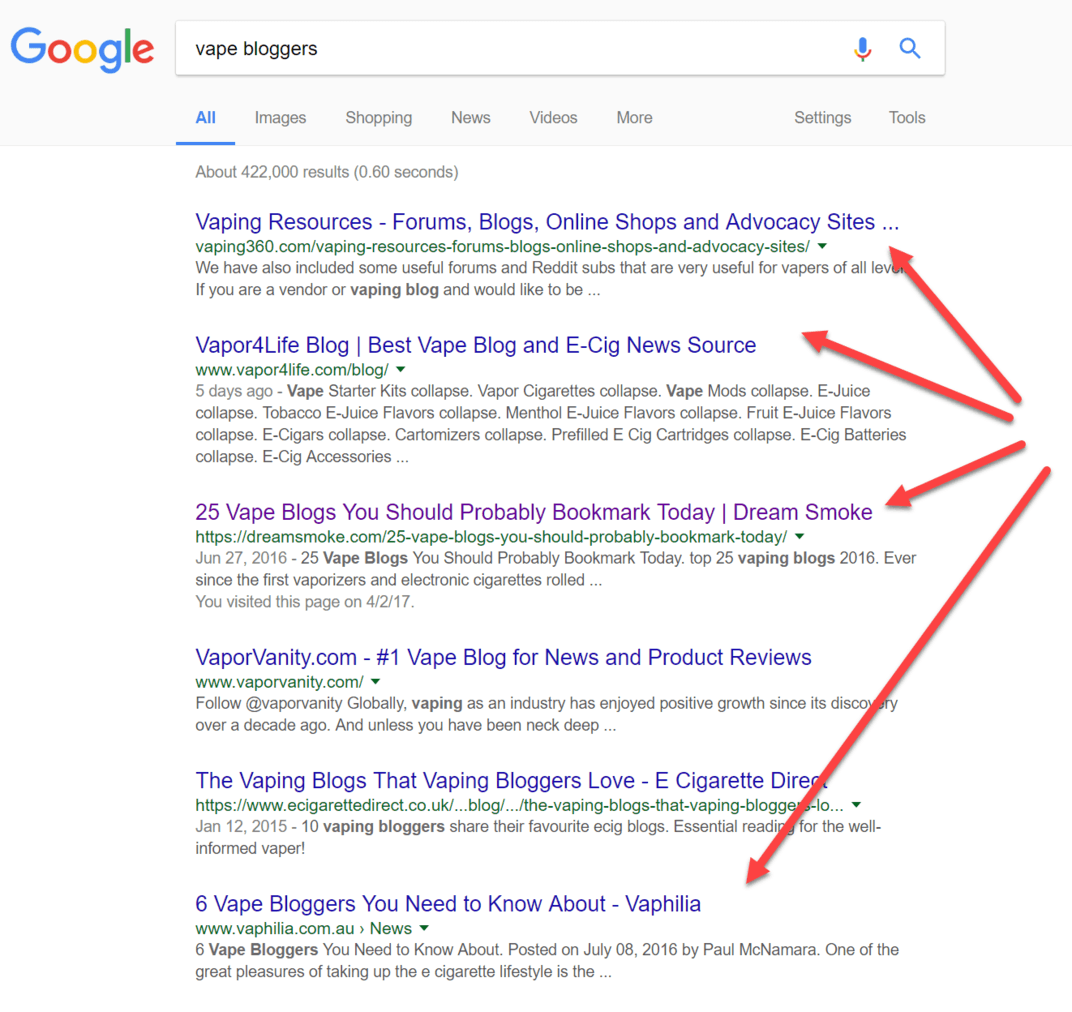The image depicts a Google search results page. The search term "vape bloggers" is entered into the Google search bar. Below the search bar, there are six clickable links associated with vaping resources and blogs, indicated in dark blue text. The colorful Google logo is prominently displayed at the top of the page, with letters in the iconic colors: a blue "G," a red "O," a yellow "O," a small blue "g," a green "l," and a red "e."

The search results include:
1. **Vaping resources, forums, blogs, online shops, and advocacy sites**.
2. **Vapor for Life blog**.
3. **Vape best, best vape blog, and e-cig news source**.
4. **25 vape blogs you should probably bookmark today**.
5. **VaporVanity.com, the number one vape blog for news and podcast reviews**.
6. **The vaping blogs that vaping bloggers love, from eCigarettesDirect**.
7. **Six vape bloggers you need to know about**.

These results are aimed at directing users to various blogs, forums, and resources related to vaping, providing information, news, reviews, and recommendations within the vaping community.